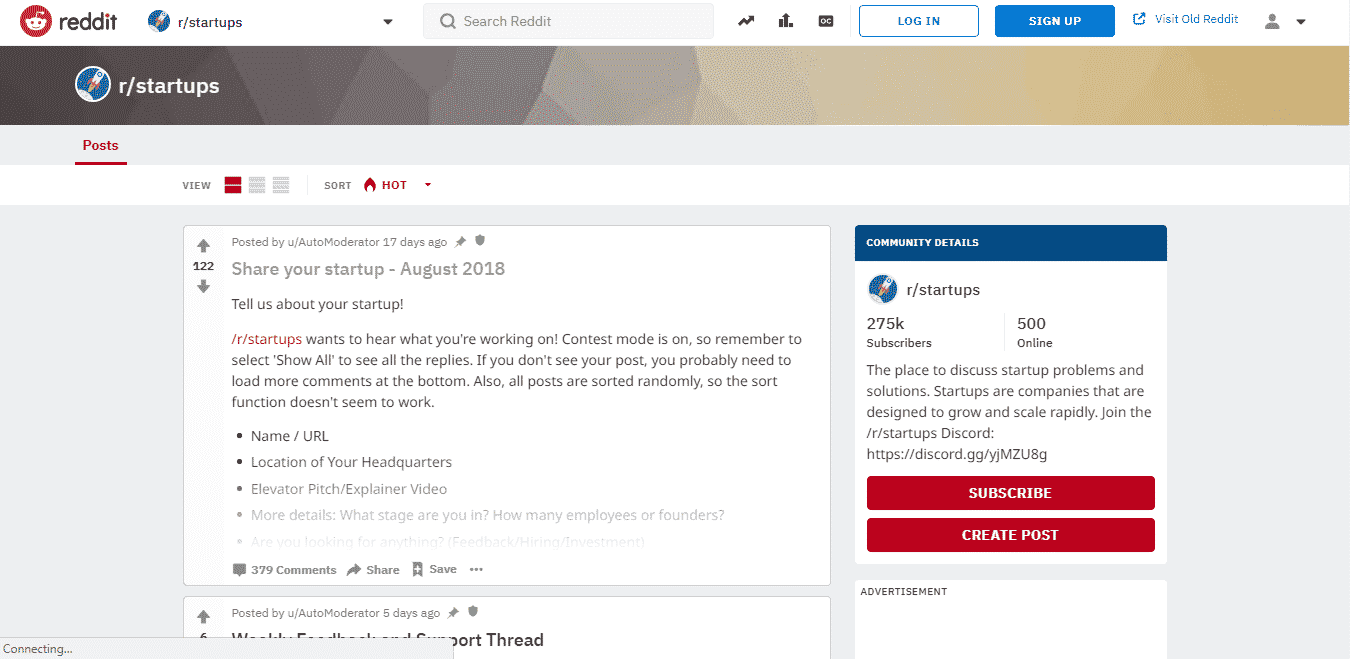"Screenshot of the r/startups subreddit main page. The top section features the Reddit logo, search bar, and options for 'Login' and 'Sign Up,' with 'Login' displayed in a white rectangle with blue text and 'Sign Up' in a blue rectangle with white text. Below the header, there are prompts to 'Visit Old Reddit' and further options related to the subreddit, including 'r/startups,' 'Post,' 'View,' 'Sort,' and 'Hot.' Community details indicate that r/startups has 295k subscribers, about 500 of whom are currently online. The subtitle reads, 'The place to discuss startup problems and solutions. Startups are companies that are designed to grow and scale rapidly.' There is an invitation to join the r/startups Discord with an accompanying link. Lastly, a prominent red rectangle with 'Subscribe' in white text and another red rectangle beneath it with 'Create Post' in white text conclude the interface."